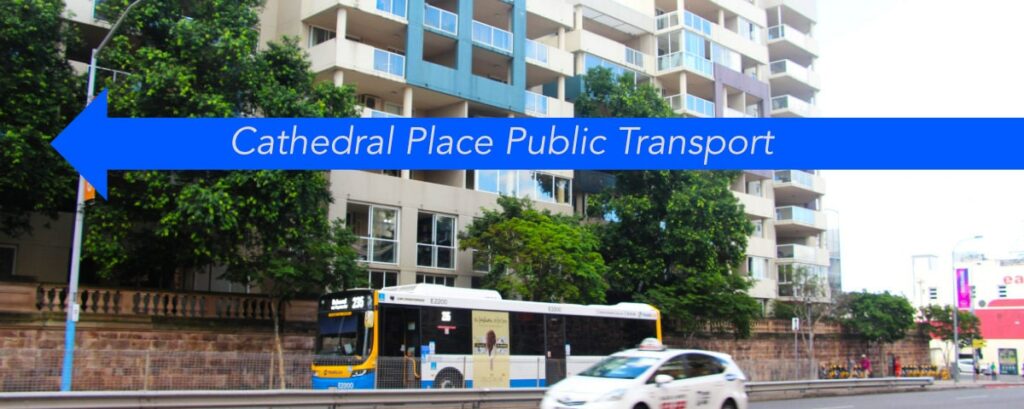The image captures a vibrant urban scene featuring public transportation. Dominating the setting is a white, blue, and yellow city bus driving from right to left, with a white hatchback, likely a taxi, adjacent to it. Both vehicles feature unreadable text. Central to the composition is a prominent blue arrow pointing to the left, superimposed with the text "Cathedral Place Public Transport." This arrow spans the breadth of the image. In the backdrop stands a multi-story apartment building with white and blue accents, fronted by a stone wall and lush trees. To the right edge of the image, a shop with a visible street light in the vicinity adds to the bustling atmosphere.